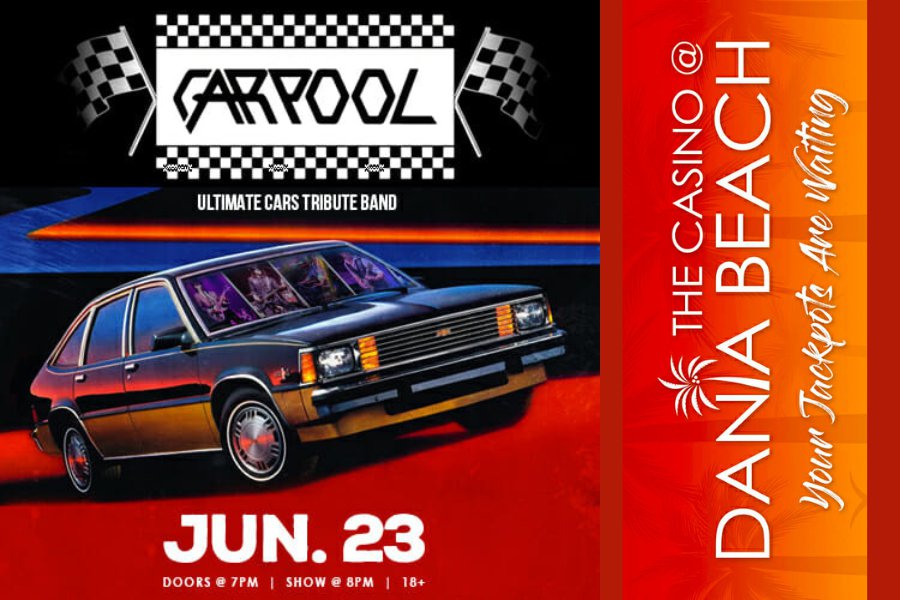The horizontally aligned rectangular poster prominently features an advertisement for the Ultimate Cars Tribute Band. The centerpiece of the poster is a vintage car positioned at a slanted angle, revealing its front end and right side. Above the car, there is a striking black background with a rectangular white banner that reads "CARPOOL" in all caps, tilted slightly for emphasis. This banner is framed by black and white checkered rectangles and flanked by two checkered racing flags on the left and right. Directly below "CARPOOL," the text reads "Ultimate Cars Tribute Band."

Beneath the car, bold white letters spell out "JUN. 23" with additional, smaller text providing event details: "Doors: 7 p.m. Show at 8 p.m. 18+." The right side of the image features a vertical, white, all-caps text that reads "DANIA BEACH," with a unique design element where the dot of the "I" is replaced by palm leaves. Above this vertical text, it says "The Casino at Dania Beach," followed by the tagline "Your jackpots are waiting." The entire right side of the poster, as well as the area beneath the car, is colored in a warm, reddish-orange background.